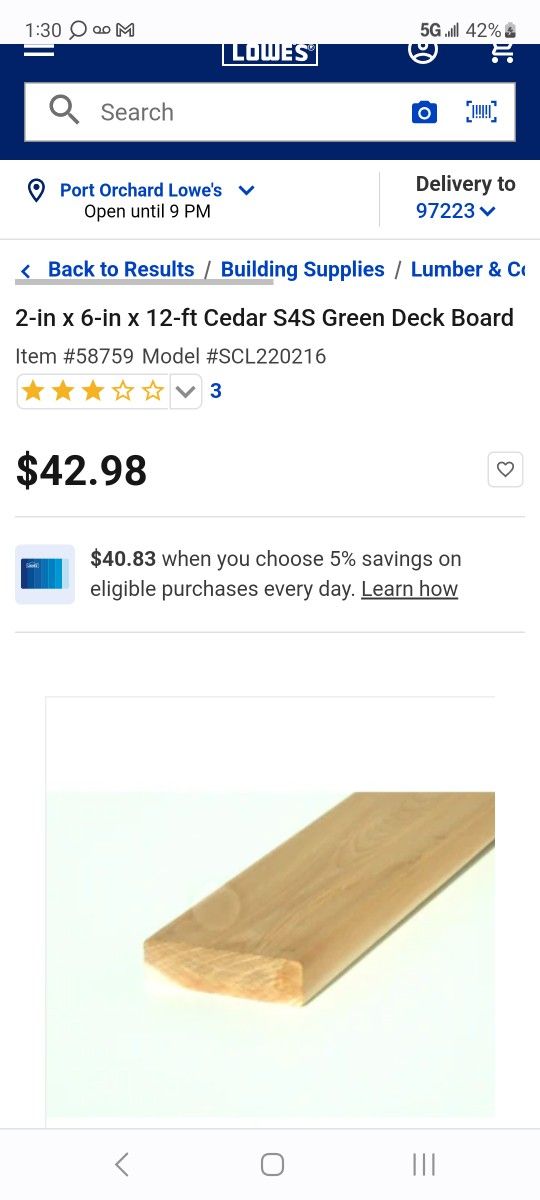This image depicts a screenshot of a phone interface displaying a product listing from Lowe's website for 2x6x12-foot cedar S4S green deck boards.

At the top left of the screen, the time is indicated as 1:30, next to a search icon, two circles, and the Microsoft Outlook logo. On the upper right, the indicators show 5G connectivity, a Wi-Fi icon, and battery life at 42%.

The main content is structured under a dark blue header featuring an outline image of a person's head and shoulders, the white Lowe's logo centered within its distinct shape, and another person icon next to a shopping cart.

Beneath the header, a white search bar with a magnifying glass icon and the word "Search" to the left and a blue camera icon is displayed. Below this is a location descriptor "Port Orchard, Lowe's" with a blue dropdown arrow, noting the store is open until 9 p.m.

A gray line separates this from the next section, indicating delivery details to zip code 97223. Another gray line follows, introducing a navigation prompt to return to search results: "back to results / building supply / lumber."

The product title "2 inch x 6 inch x 12 foot cedar S4S green deck boards" is displayed in bold black font, followed by its item number 58759 and model number SCL220216.

Star ratings show three filled stars out of five, next to a "3" in blue font. The price is marked as $42.98 with a heart icon beside it for saving the item. Below this, a promotional offer is described, "Save $40.83 with 5% savings on eligible purchases every day. Learn how" underlined.

The next section features a product image on a light green background with a brown wooden board, separated by a gray line and accompanied by navigation icons below: a back arrow, a rounded circle, and a menu icon with three vertical lines.

This detailed caption aims to provide a comprehensive textual representation of the image's content and layout.